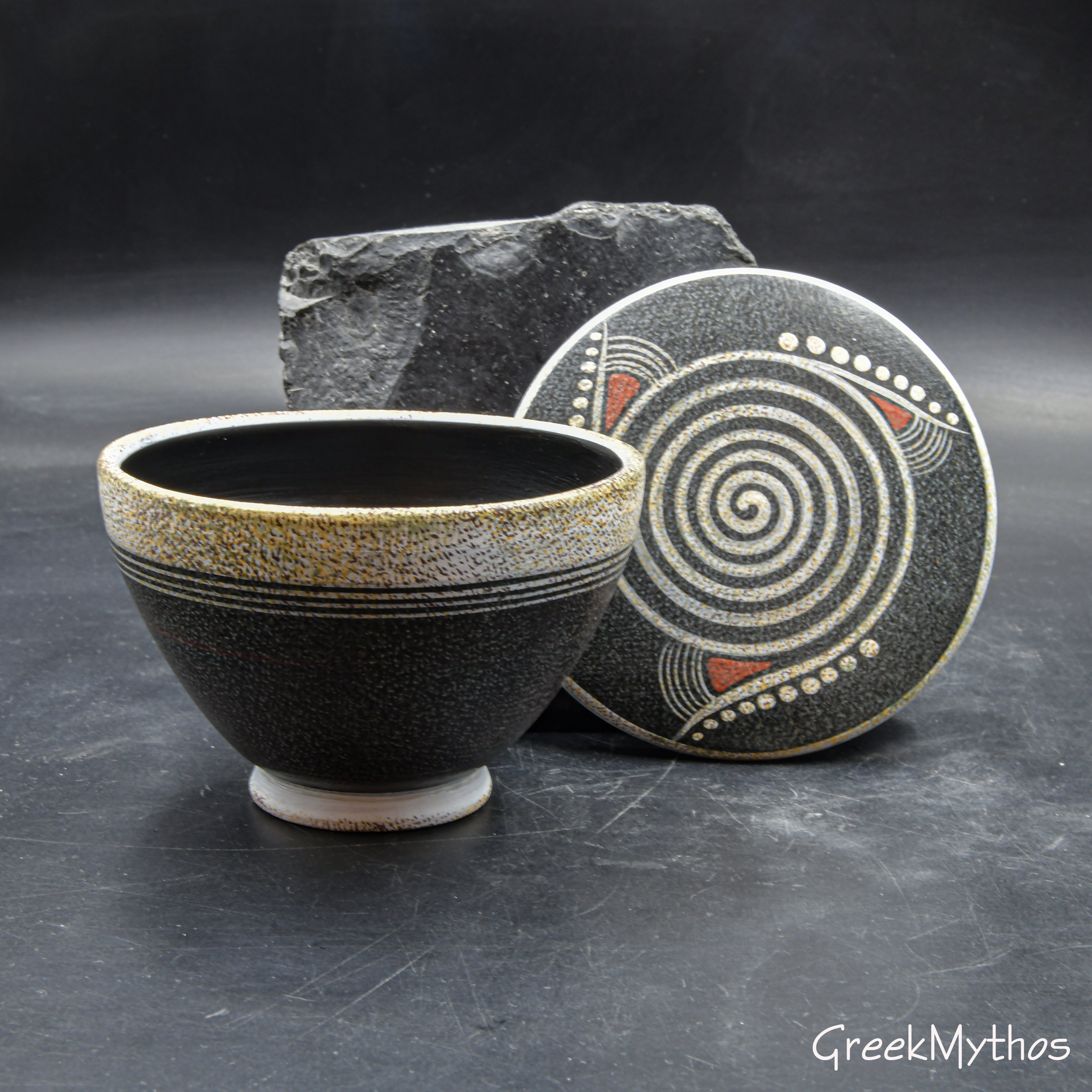In the image, there is a piece of Greek pottery set against a monochromatic background. The main focus is a ceramic bowl with a narrow base and a wide mouth, featuring a dark gray bottom and a white foot. The top of the bowl is predominantly white. Accompanying the bowl is an intricately designed lid propped against a dark, cool-looking rock, possibly to enhance the composition. The lid showcases a large, multi-layered spiral with abstract accents and cat ear-like triangular designs outlined in gold and filled with red and gold detailing. The bowl and lid are situated on a surface that appears to be a marble slab, and the overall color palette includes shades of black, dark gray, and white. At the bottom right corner of the image is a watermark or logo reading "Greek Mythos," indicating that the items are likely related to Greek mythology and culture.